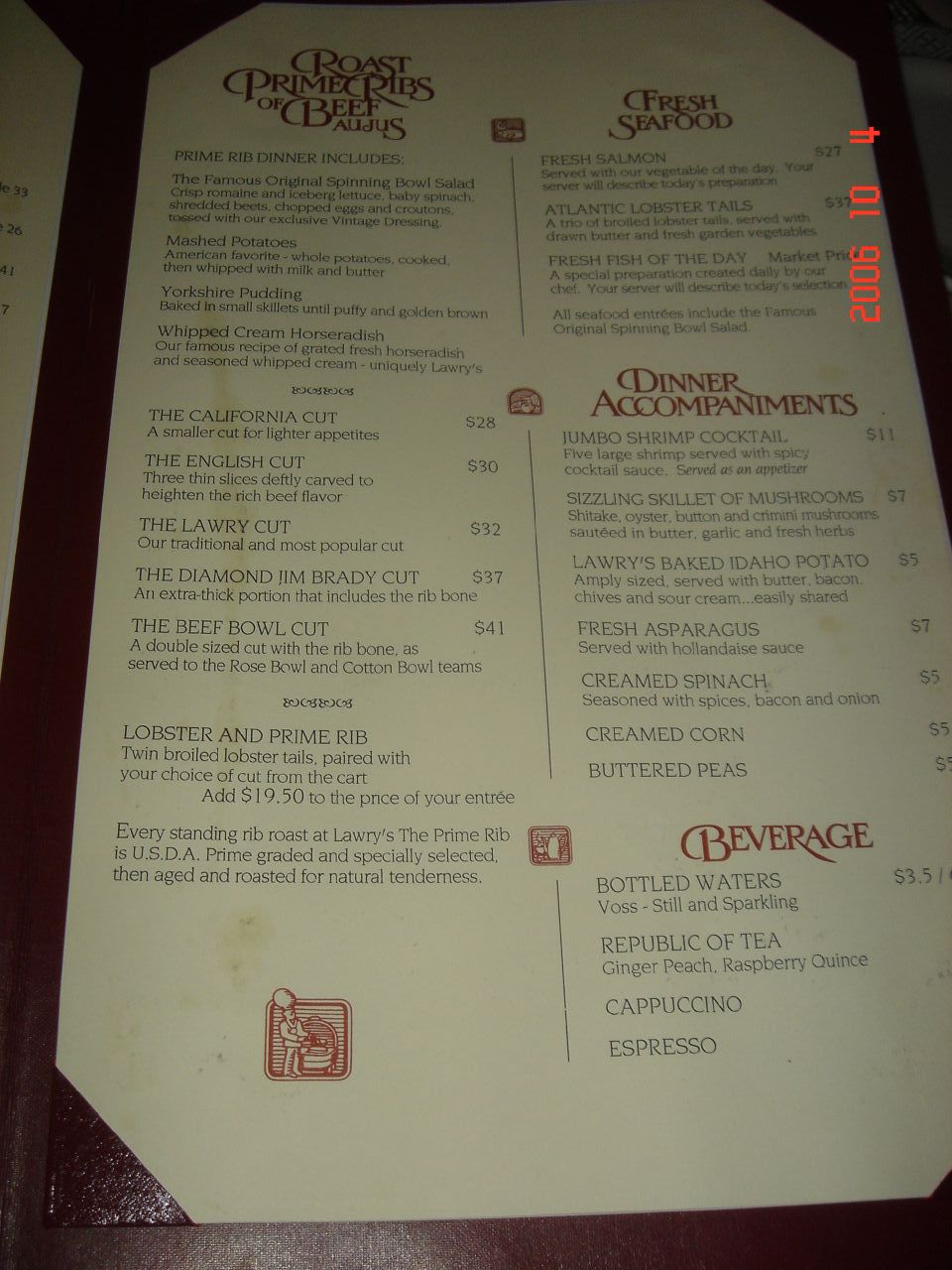This photograph showcases a restaurant menu set against a pristine white background, featuring an elegant dark brownish border. The menu's text is artistically rendered in a combination of red and black hues. The menu is thoughtfully divided into two distinct sections at the top.

On the left side, the top section is headlined with "Roast Prime Ribs of Beef." Directly beneath this title, various sumptuous options are listed, including Yorkshire pudding and whipped cream horseradish. Following these delicacies, a range of different beef cuts is detailed: the California Cut, the English Cut, the Lowry Cut, and the Beef Bowl Cut. The section concludes with the tempting option of "Lobster and Prime Rib."

The right side of the menu begins with a bold red heading proclaiming "Fresh Seafood," followed by three enticing seafood options. Below this, another red header introduces the "Dinner Accompaniments" category, featuring selections like Jumbo Shrimp Cocktail, Sizzling Skillet of Mushrooms, Fresh Asparagus, Creamed Spinach, Creamed Corn, and Buttered Peas. At the bottom of this section, "Beverages" is also highlighted in red, offering four drink choices to complement the meal.

This detailed menu promises a fine dining experience with a variety of indulgent options to satisfy any palate.